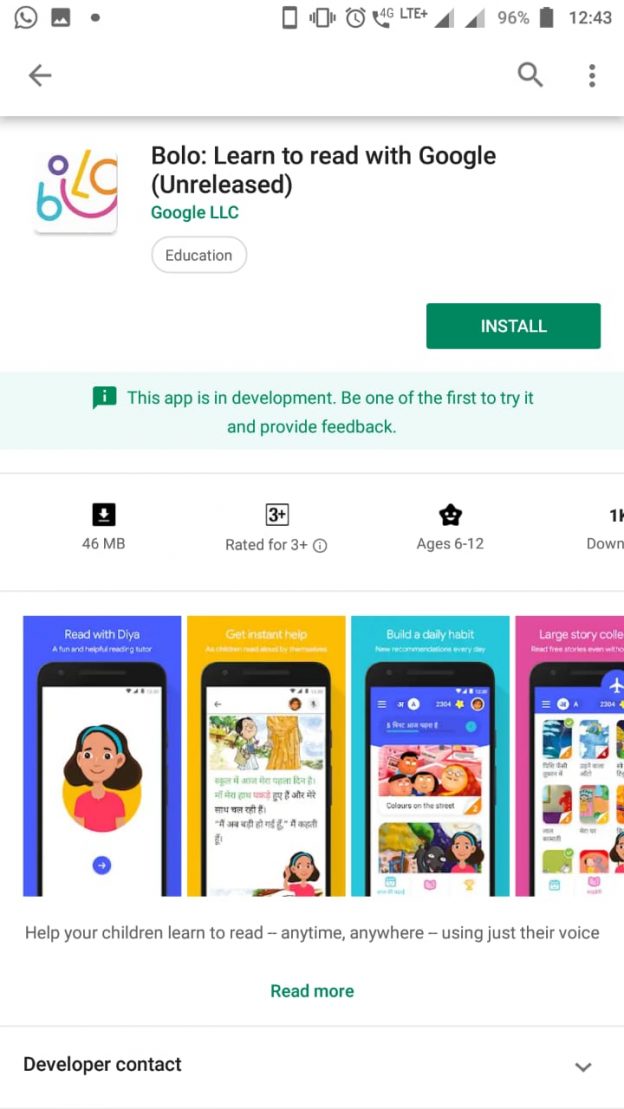The image showcases a mobile phone screenshot of an app page for an unreleased Google LLC education application named "Bolo: Learn to Read with Google". The top of the screen displays the app's name alongside the label "Google LLC Education" and an "Install" button in the bottom-right corner of this section. The page indicates that the app is still in development with a call to action inviting users to be among the first to try it and provide feedback.

The app details reveal that it is 46 MB in size, rated for ages 3 and up, and specifically designed for children aged 6 to 12. Highlighted features include "Read with Dalia," which offers instant help, "Build a Daily Habit," and a "Large Story Collection." The description emphasizes that it helps children learn to read anytime, anywhere, using their voice.

At the bottom of the image, there is a clickable "Read More" option in teal, and a "Developer Contact" section with a down arrow icon for additional information. The status bar at the top of the screen shows the time as 12:43, with the battery at either 60% or 96% charged, along with other standard notification icons.